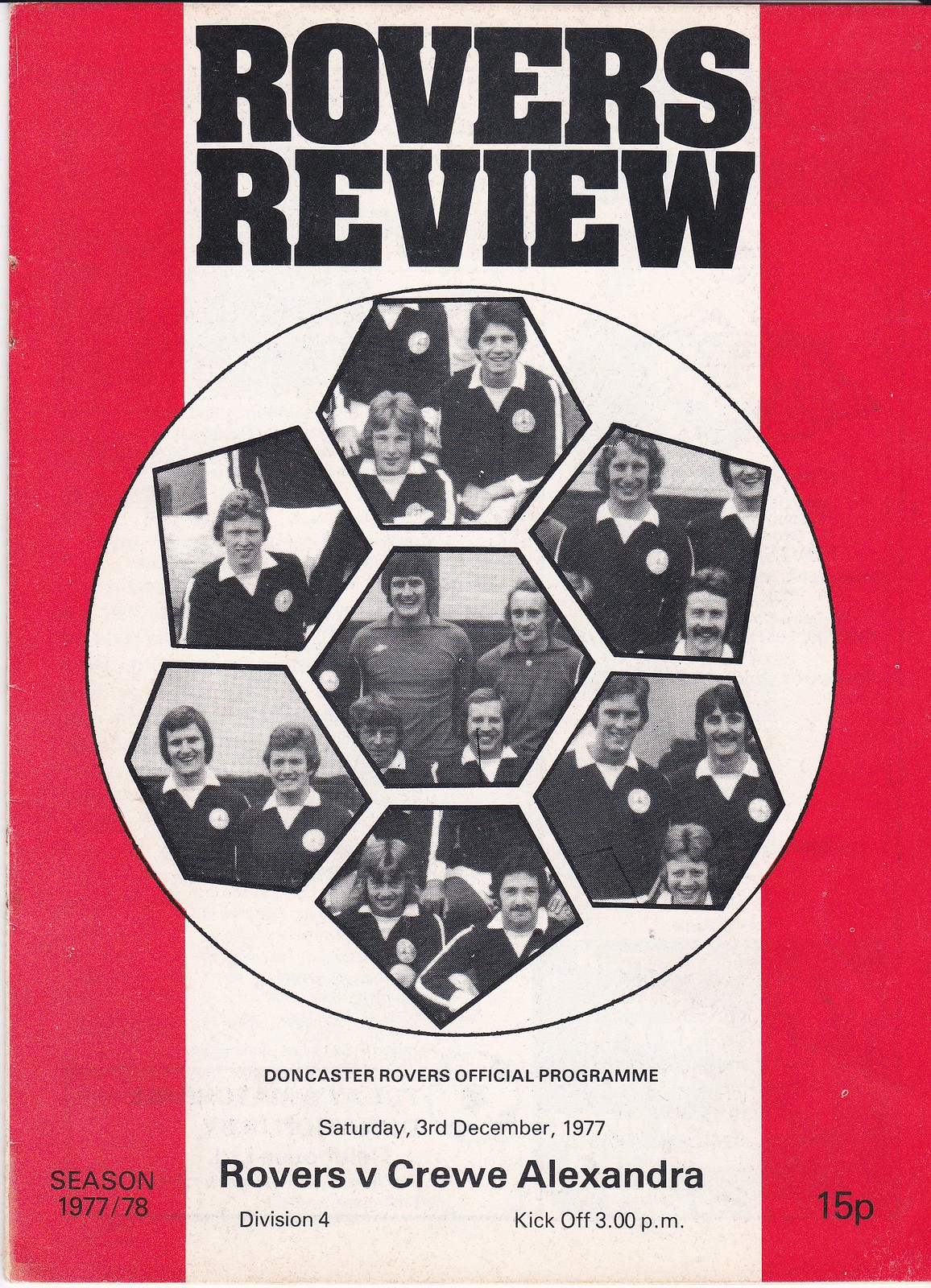The image depicts the cover of a football program from December 3, 1977. The design features a prominent white stripe running vertically down the center, flanked by bold red stripes on both sides. At the top of the cover, in large black capital letters, is the title "Rovers Review." Central to the design is a circular motif resembling a soccer ball, with pentagonal and hexagonal frames inside it containing black-and-white photographs of players from the Doncaster Rovers team, who are seen wearing white-collared jerseys with dark and white stripes. Below this imagery, the text reads: "Doncaster Rovers Official Program. Saturday, 3rd December, 1977. Rovers vs. Crewe Alexandra. Division IV, Kickoff 3pm. Season 1977-78." In the bottom right-hand corner, the price is noted as "15 pence."